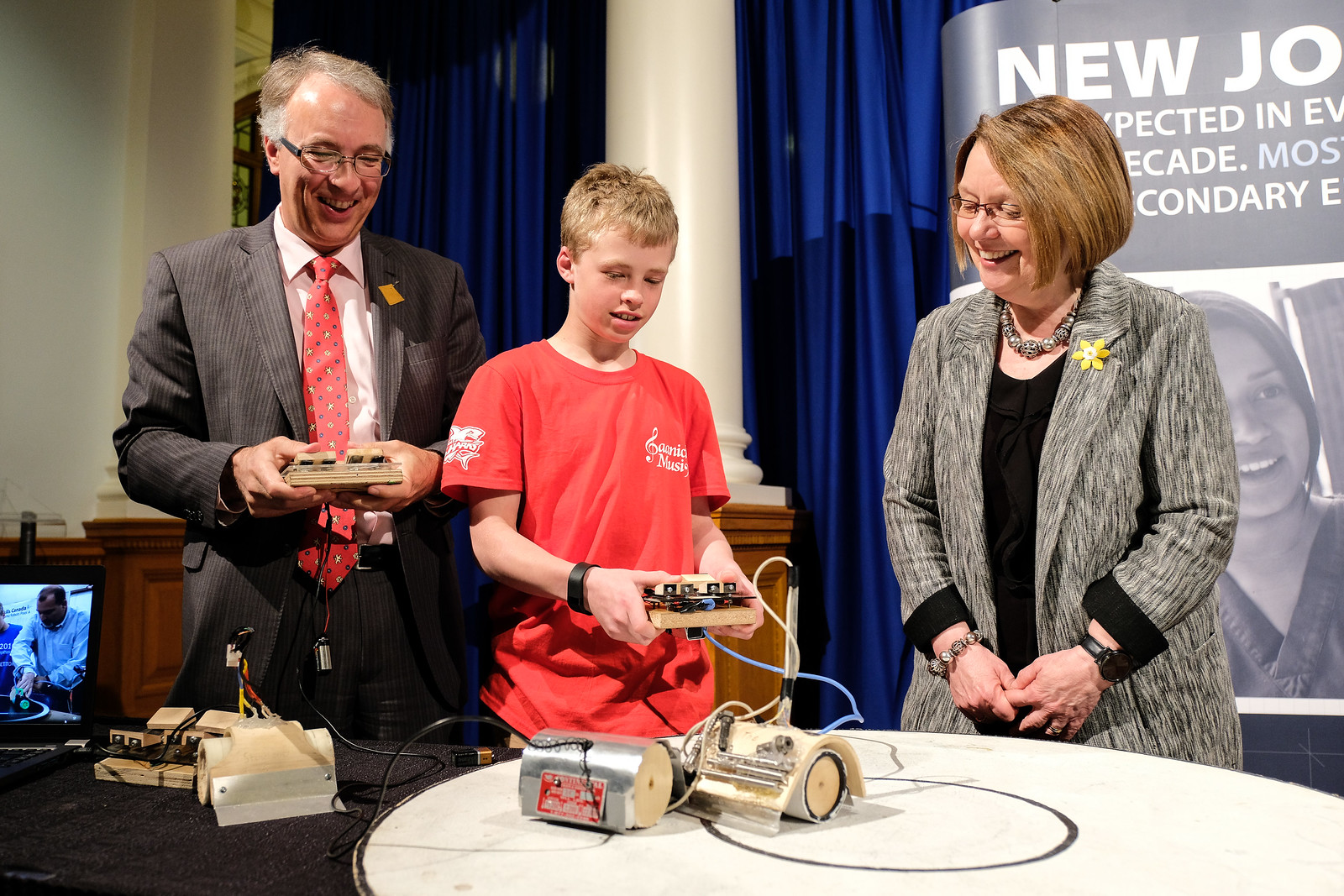In the image, a young blonde Caucasian boy stands in the center, proudly holding a wooden electronic device with various buttons, wires, and "gigaws" extending from it, connected to large batteries on a circular table. The boy, wearing a red t-shirt with white lettering and a black wristband, appears to be demonstrating his science project. To the right, a delighted middle-aged Caucasian woman with chin-length hair, wearing spectacles, a two-toned black and white blazer with a yellow flower pin, a silver necklace, a long-sleeved black dress, a bracelet, and a wristwatch, gazes at the boy. To the left, a tall middle-aged man with gray hair, large black-rimmed glasses, a pinstriped suit, and a red tie, holds a similar device, grinning widely. Behind this trio, a screen on the far left shows an image of a man of color wearing a blue shirt, possibly engaged in a similar activity. In the background, blue curtains, a white pillar, and a partially visible gray and white poster can be seen, with words like "new" and "J-O" hinting at the text "jobs expected in every decade" and an image of a woman's face at the bottom.